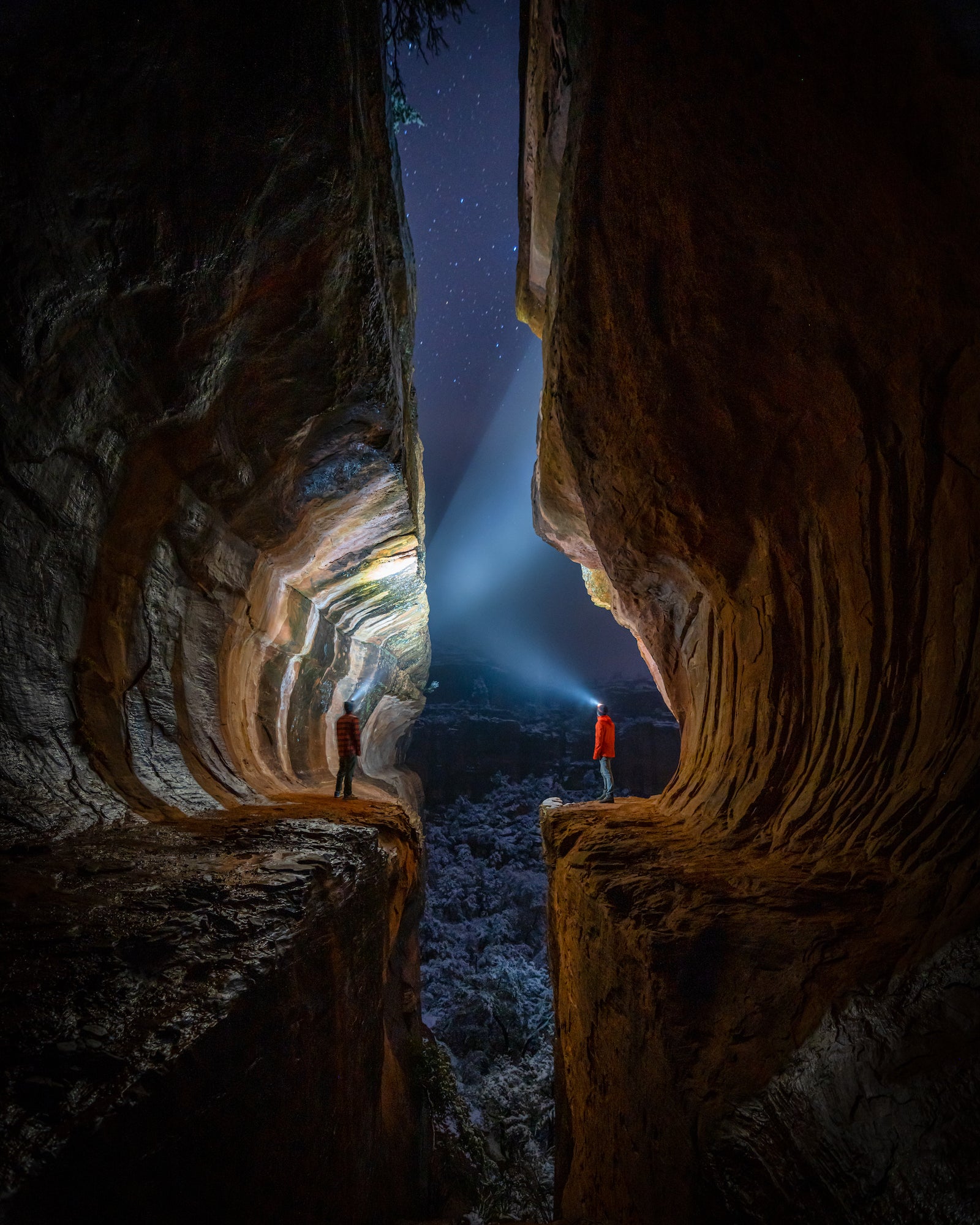The image appears to be a highly detailed and creative animated illustration, possibly from a book or a video game. It features a split cave scene framed within a vertically aligned rectangular format. On the left side, a person depicted as a black silhouette stands on a cliffside wearing a flannel shirt and using a headlamp, which casts light upwards toward a dark, star-speckled sky. The cliff on this side has noticeable white and gray stripes. On the right side, another individual, dressed in an orange/red jacket and dark gray or blue pants, stands in a similarly C-shaped cutout on a brown cliff. This person also wears a headlamp, their light directed at the opposite cliff. The scene includes a rocky gap at the bottom and a night sky filled with stars above, framed by vertical cliffs on either side. The overall ambiance is one of exploration within a beautifully illustrated, surreal landscape.